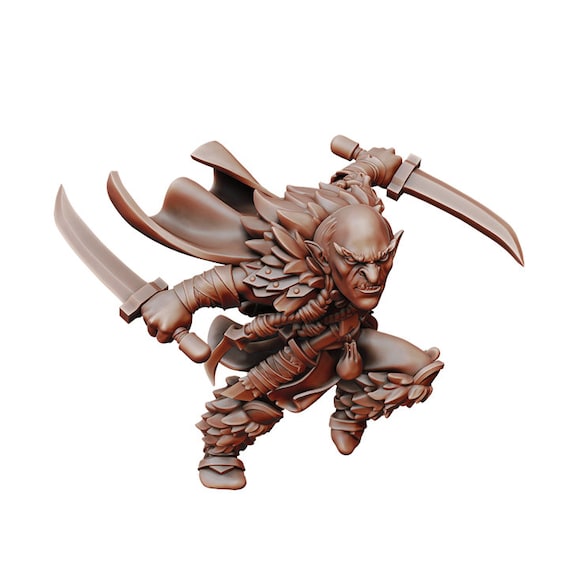The image depicts a detailed sculpture or digital illustration of a villainous, fantasy character, entirely rendered in brown. The character features a round, bald head and a face with a menacing expression, marked by mean eyes, pointy eyebrows, a prominent pointy nose, and grizzled teeth. His ears taper to points at their ends. His body is short, stout, and armored with what appears to be leaves and feathers covering his knees, shins, and wrists, suggesting protective gear. The character's arms are outstretched to both sides, each hand gripping a curved sword—one pointed backwards on the left and one pointed forward on the right. He is posed in a dynamic, lunging stance, with one knee bent forward to the right and the other leg extended back to the left, which is the only foot touching the ground. He wears boots with additional feathering but no pants, and a billowing brown cape flows behind him. The entire scene is set against a stark white background, giving it a striking, three-dimensional appearance.